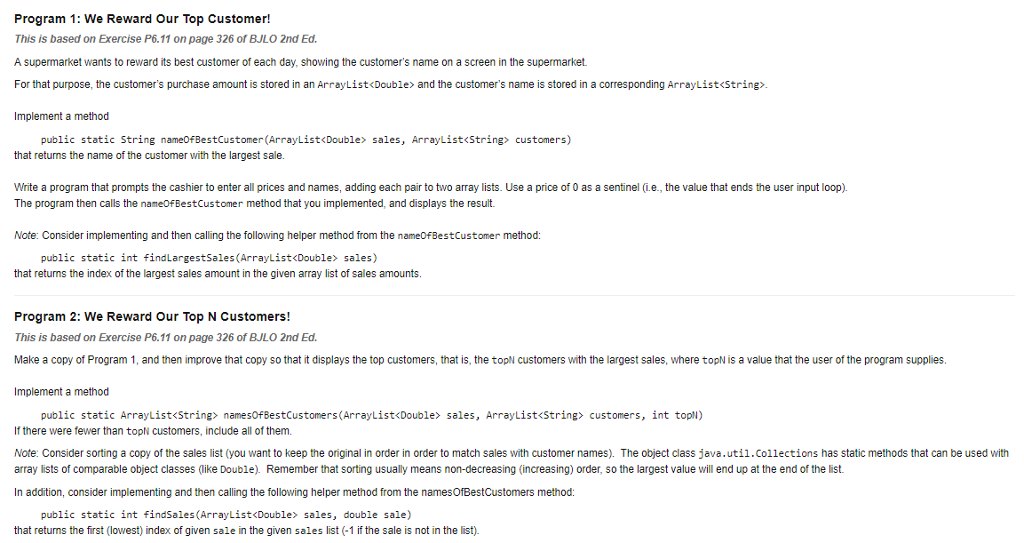**Detailed Caption:**

The image features a section from an instructional textbook set against a white background, detailing two programming exercises aimed at rewarding top customers in a supermarket setting. 

**Program 1 - Rewarding the Top Customer:**
Based on an exercise from page P611 (BJLO, 2nd edition, page 328), this program is designed to reward the best customer each day by displaying their name on a screen in the supermarket. To achieve this, the customer's purchase amount is stored in an ArrayList of type Double, and their name is stored in a corresponding ArrayList of type String. The program includes the definition of a method `public static String nameBestCustomer(ArrayList<Double> sales, ArrayList<String> customers)` that returns the name of the customer with the highest purchase amount. The program prompts the cashier to enter prices and names, adding each pair to the respective ArrayLists. A price of 0 cents is used to signify the end of input.

**Program 2 - Rewarding the Top N Customers:**
Based on an exercise from page 11 (BJLO, 2nd edition, page 326), this exercise expands on Program 1. It instructs users to make a copy of the initial program and modify it to display not just the top customer, but the top N customers with the largest sales, where N is a value provided by the user. The implementation includes writing a new method to determine and display the top N customers, along with additional text explaining how to implement the relevant code changes.

The image contains substantial text explaining the steps, methods, and code structure needed to complete both programming tasks.